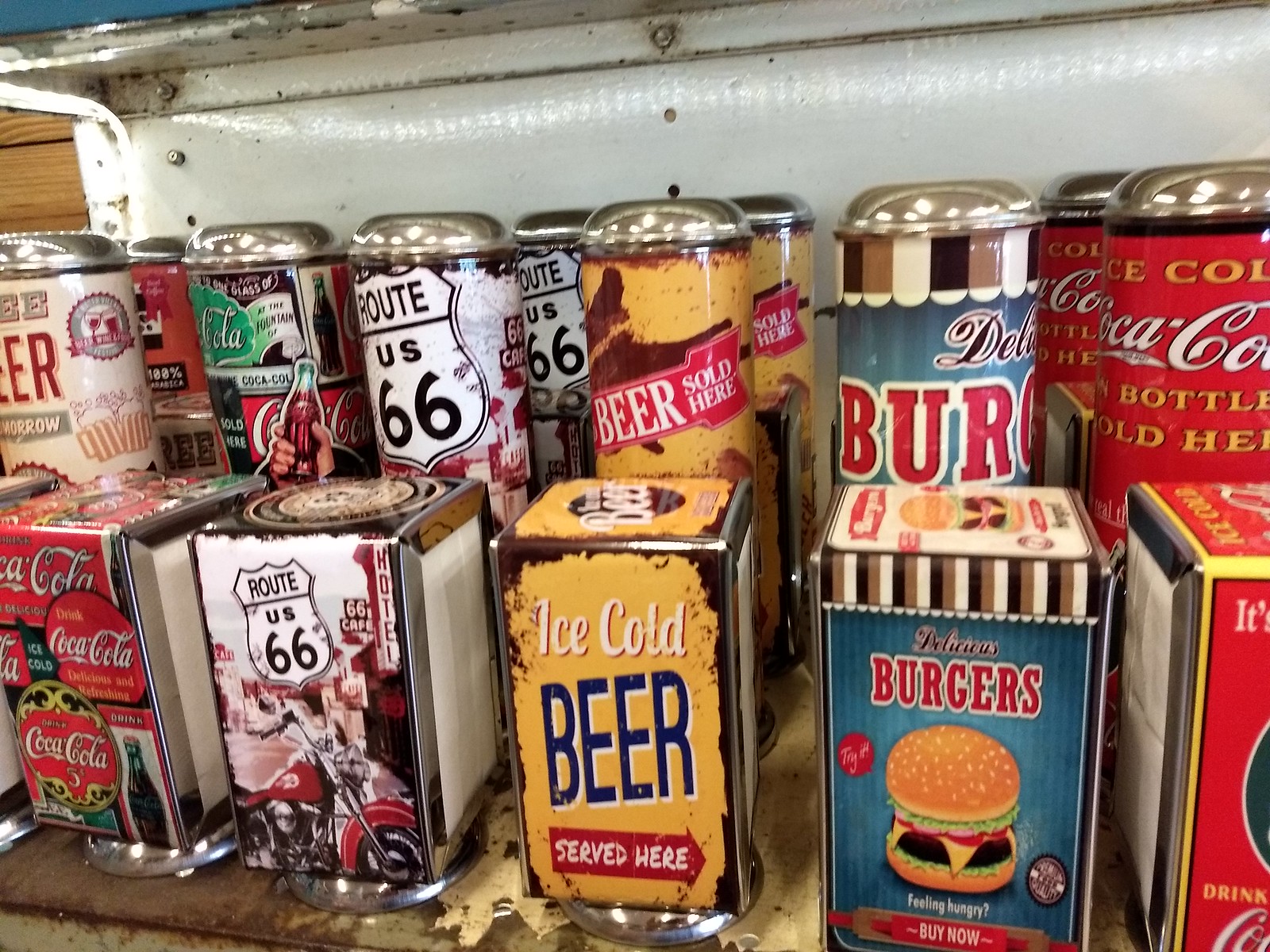The image depicts the inside of a rustic, possibly vintage-themed refrigerator or cooler, likely reminiscent of an old-timey restaurant display. At the top, there's a white metal bar with a couple of screws in it, and everything is set on a rusted metal platform. In the foreground, prominently arranged, are a series of metal napkin dispensers, each adorned with different nostalgic designs. From left to right, the first dispenser is themed with the Coca-Cola logo repeated prominently. Next to it is a Route 66 dispenser featuring a motorcycle graphic. In the middle, there's a yellow dispenser with a rustic look, bearing the words "Ice Cold Beer Served Here." To its right, another dispenser promotes "Delicious Burgers" with an image of a burger and phrases encouraging purchase and trying it out. Another Coca-Cola-themed dispenser is positioned further to the right. 

Behind these dispensers are matching cylindrical canisters or containers with lids, each corresponding to the design of the napkin dispensers in front of them. These larger metal tubes, with silver caps, align perfectly with the motifs of the napkin dispensers, adding to the cohesive and nostalgic feel of the display. The backdrop includes elements like a secondary white shelf, some wood paneling, and a blue wall in the upper left, further enhancing the vintage ambiance of the scene.